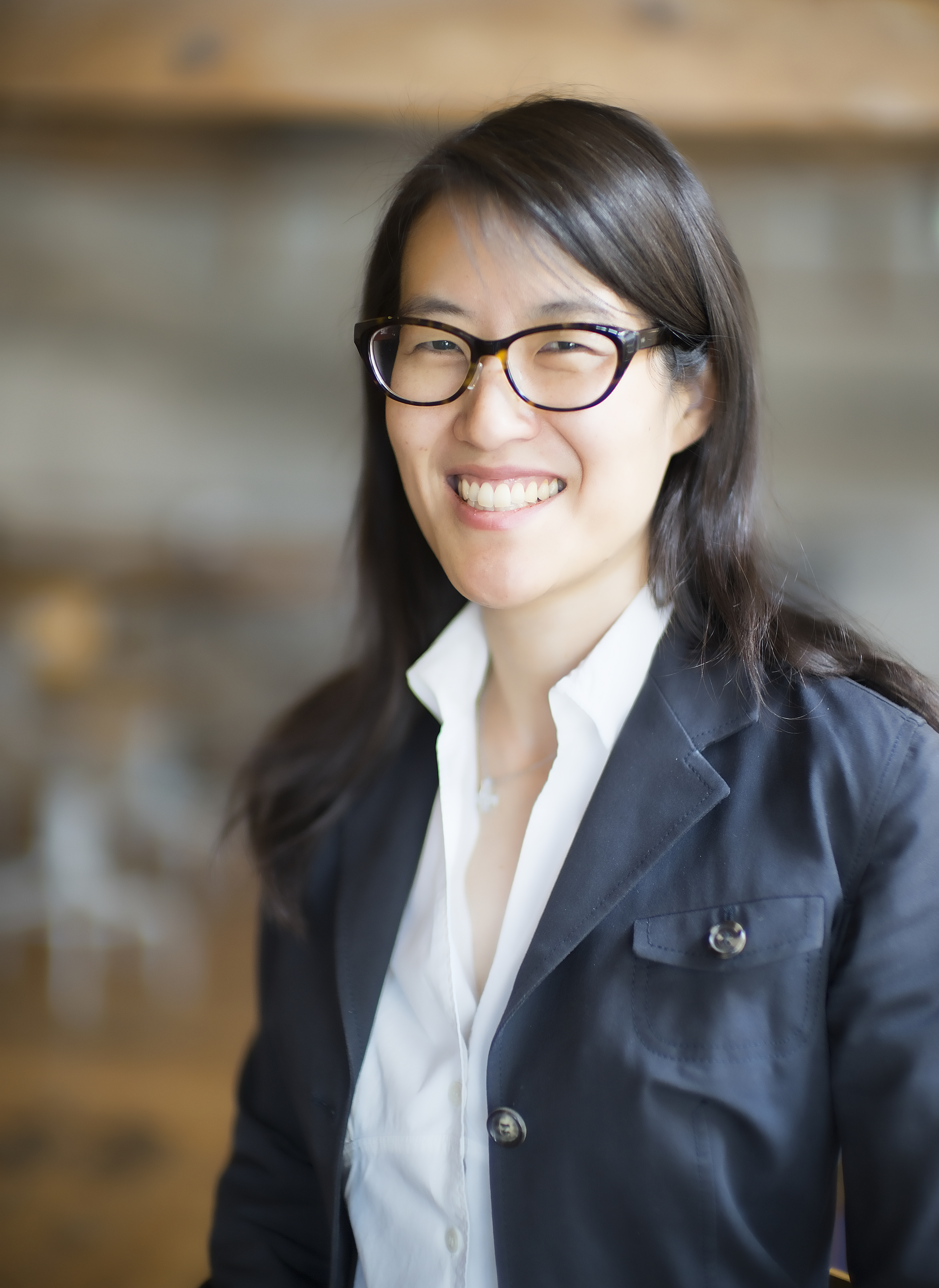A high-resolution promotional photo features a distinguished woman standing in front of a background that transitions from a creamish white at the top to gray, with a hint of green in the bottom left corner, suggesting a possible outdoor setting near a building and grassy area. The focus is on a woman of Asian descent with long, shoulder-length black hair. She is adorned in thick-rimmed black glasses, a radiant smile showcasing her white teeth, and a slightly pointed chin. She is dressed in an open white button-down shirt, paired with a grayish navy blue jacket. This image likely portrays Dr. Lisa Su, the President and CEO of AMD, a leading computer chip and software company.